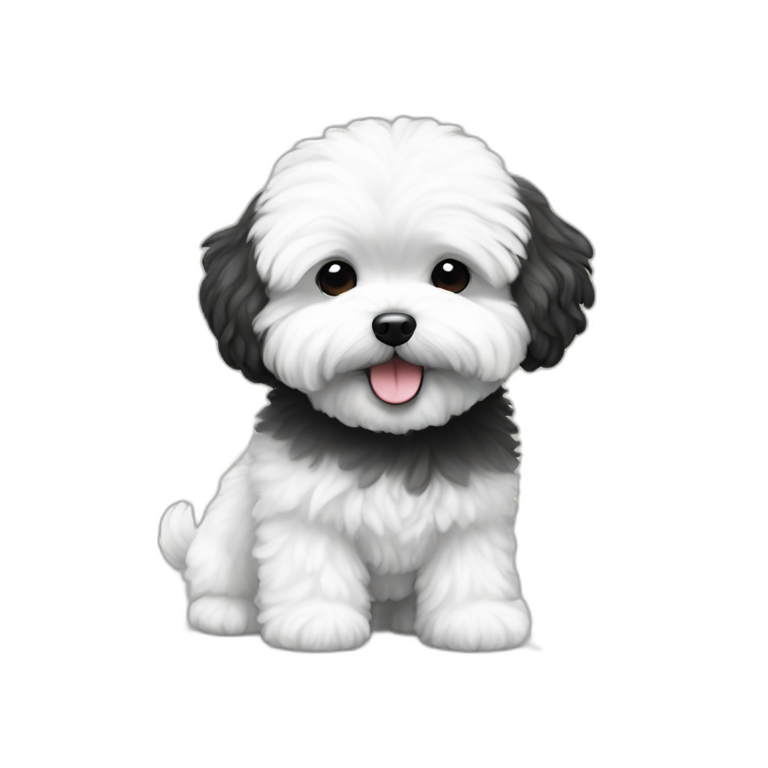This is a cartoon-style image of an adorable small puppy. The little dog, drawn in an emoji-like fashion, has primarily white fur, giving it an exceptionally fluffy and soft appearance, reminiscent of goose feathers. The puppy's most striking features include its almost black, dark gray ears and a darker gray shading around the neckline. Its eyes are very dark brown, almost black, while its small nose is distinctly black. The puppy is looking straight ahead with a joyful expression, highlighted by its pink tongue sticking out as if it's smiling. The pup's fluffy white fur, including a short tail, accentuates its cute and cuddly look. The scene shows the puppy in a seated position on a white background, with its back paws on the ground and its front legs standing up, giving an impression of playful alertness. The white fur on the top of its head is especially fluffy, almost covering its eyes, adding to its endearing charm.